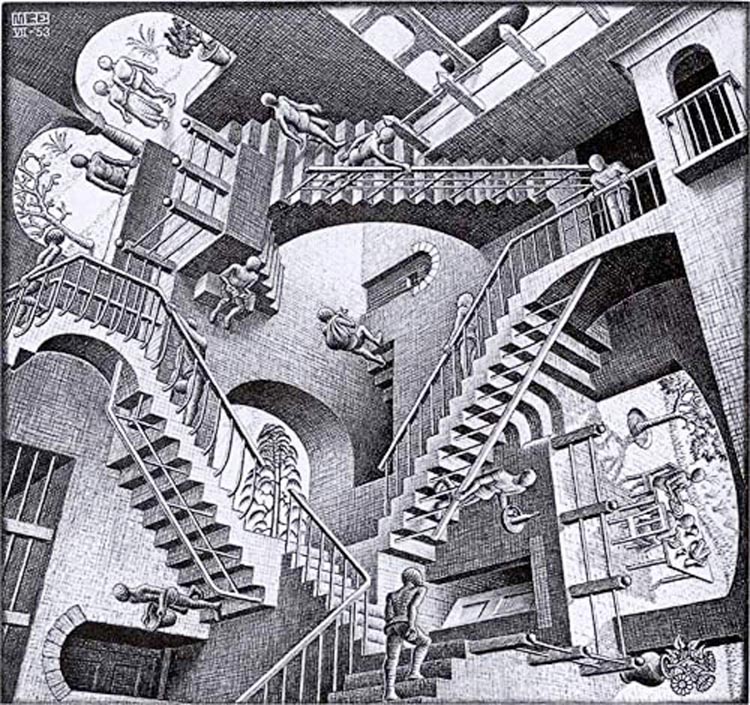This image is a famous black-and-white etching, likely by M.C. Escher, known for its mind-bending depiction of interconnected staircases. In the top left corner, the letters “M R E” appear above the Roman numerals “VII/V/3.” The etching features a series of staircases that twist and turn in impossible ways, creating an optical illusion that defies the laws of physics. The top right corner shows a light background balcony with a guardrail, which transitions into darkness through the archway.

The entire scene is populated by about a dozen human-like mannequins, faceless figures with no distinguishing features, who walk sideways, upwards, downwards, and across the various staircases. One can be seen holding a basket near a dark archway in the bottom left-hand corner, while another figure is seated at a table in the bottom right. In the bottom center, a staircase emerges with an individual climbing a flight of stairs, accompanied by a guardrail on the left side. Throughout the image, hatching and shading techniques create an illusion of depth, enhancing the surreal and abstract nature of the structure.

Overall, the intricate use of black and white, combined with great shading and multiple arcs and doors, makes this etching an intriguing, distorted visual experience that challenges the viewer’s perception of space and reality.